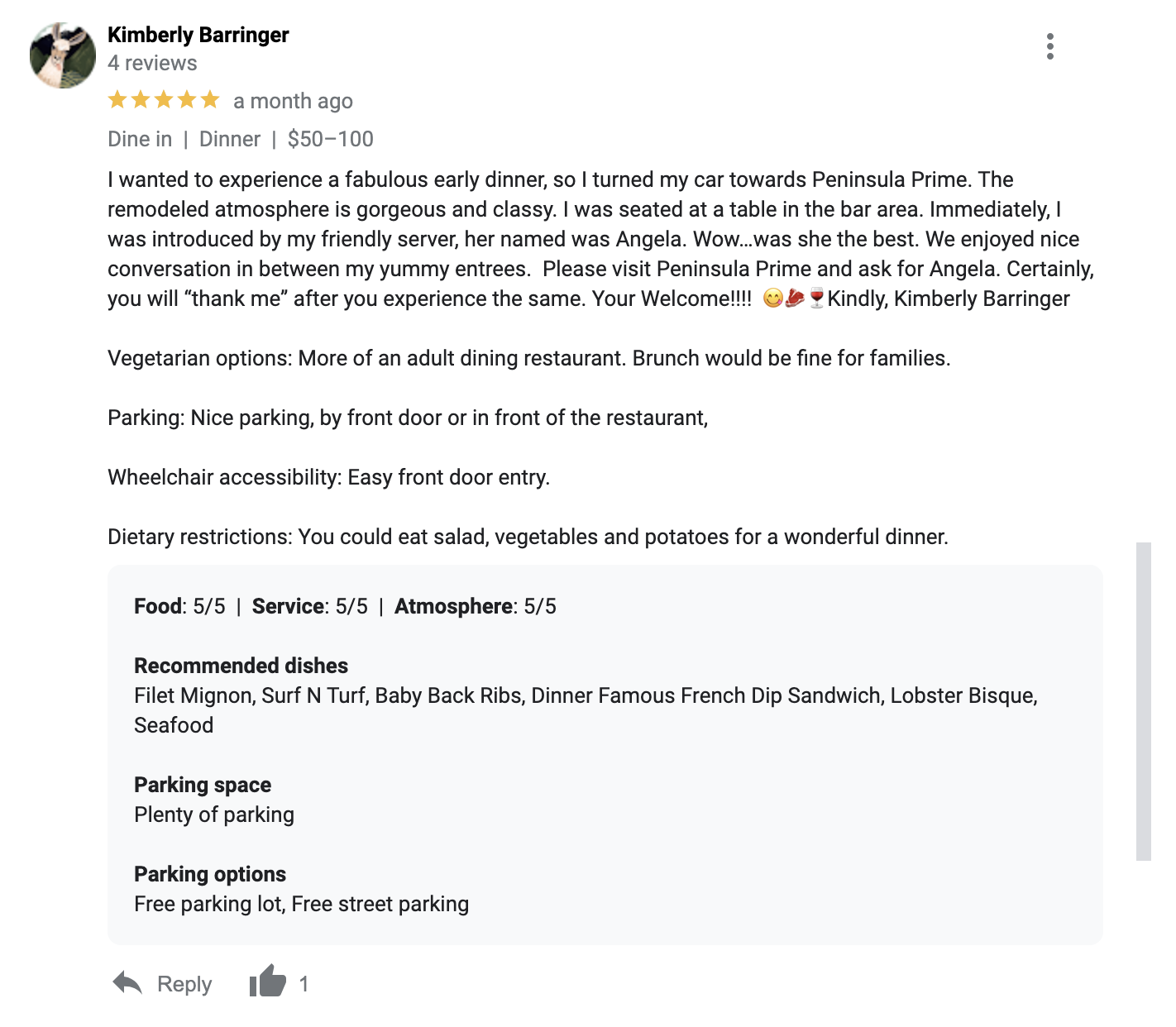**Kimberly Beringer's 5-Star Review of Peninsula Prime**

Kimberly Beringer, a reviewer with four reviews to her name, recently shared her delightful experience at Peninsula Prime, a dining venue she visited for an early dinner a month ago. She awarded the establishment a stellar five-star rating. According to Kimberly, the cost of her meal ranged from $50 to $100, and she chose to dine in for dinner.

In her review, Kimberly expresses her initial excitement to indulge in a fabulous early dinner, which led her to Peninsula Prime. Upon her arrival, she was impressed by the remodeled atmosphere, describing it as both gorgeous and classy. Kimberly was seated at a table near the bar and was immediately greeted by her friendly server, Angela. She highlights Angela's exceptional service, noting that they engaged in pleasant conversation between her enjoyment of what she describes as "yummy entrees."

Kimberly strongly recommends Peninsula Prime and specifically suggests requesting Angela as your server for an equally gratifying experience. Additionally, she points out that the restaurant offers vegetarian options and is more suited for adult dining, though brunch could be a good time for family visits. Parking is convenient, with spaces available right by the front door or in front of the restaurant. There is also wheelchair accessibility with easy front door entry.

For those with dietary restrictions, Kimberly mentions that you can opt for a meal consisting of salad, vegetables, and potatoes. 

Finally, Kimberly rates the overall food, service, and atmosphere each a perfect five out of five. She recommends several dishes including the filet mignon, surf and turf, baby back ribs, the famous French dip sandwich, lobster bisque, and other seafood options. Parking is plentiful and free, either in the parking lot or on the street.

"You're welcome in advance," signs off Kimberly Beringer, inviting others to experience Peninsula Prime and see for themselves.